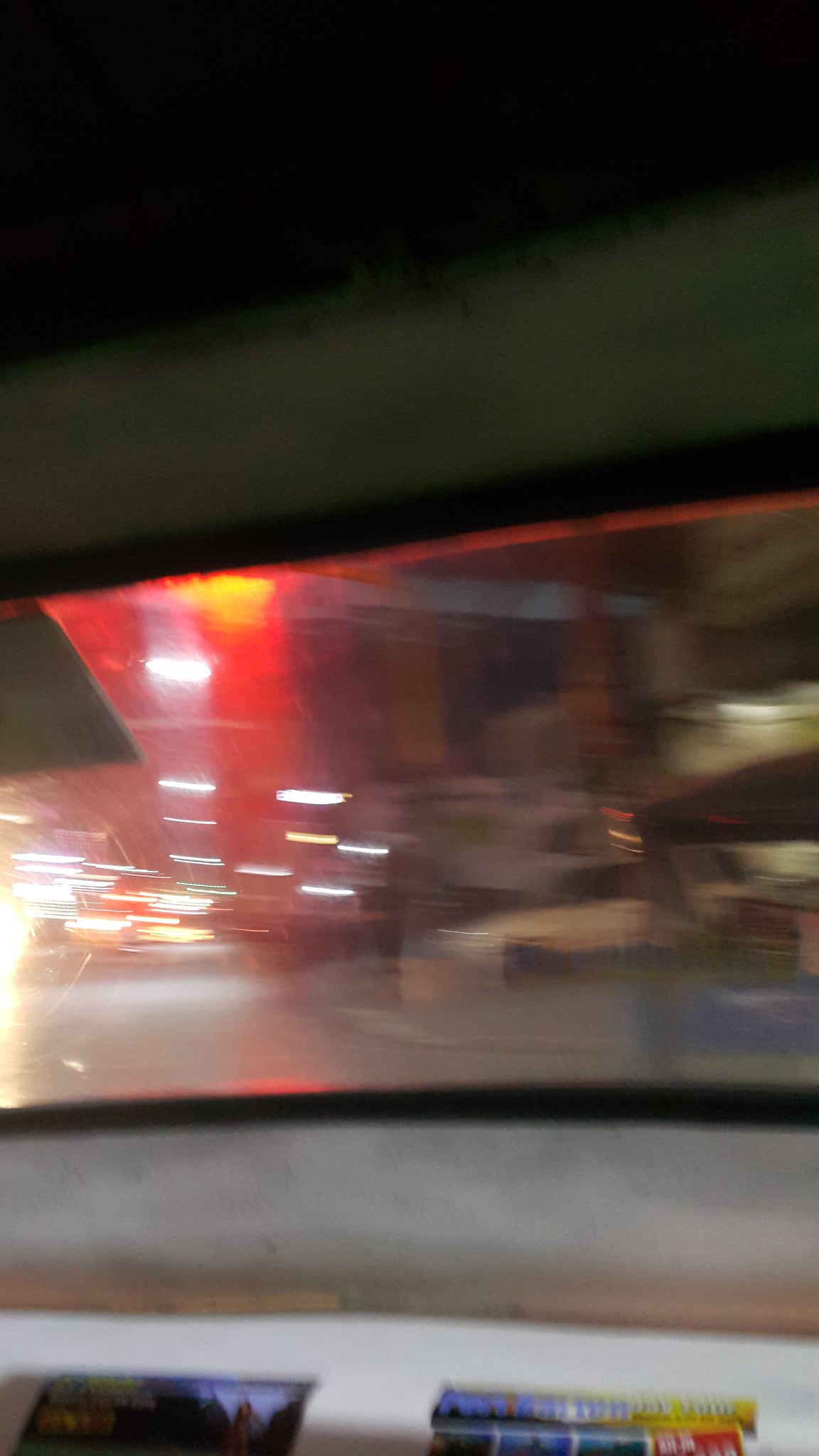The image captures a blurred view from the interior of an older, weathered vehicle, presumably a car. The minimalist and somewhat worn dashboard is visible, indicating that this is likely not a modern model. The scene appears to take place while the vehicle is stationary, evidenced by the red traffic light visible at the top of the frame. Another car is seen approaching from the side but is not in motion. On the dashboard, two packages resembling candy bars can be discerned, along with a small photograph placed adjacent to them.